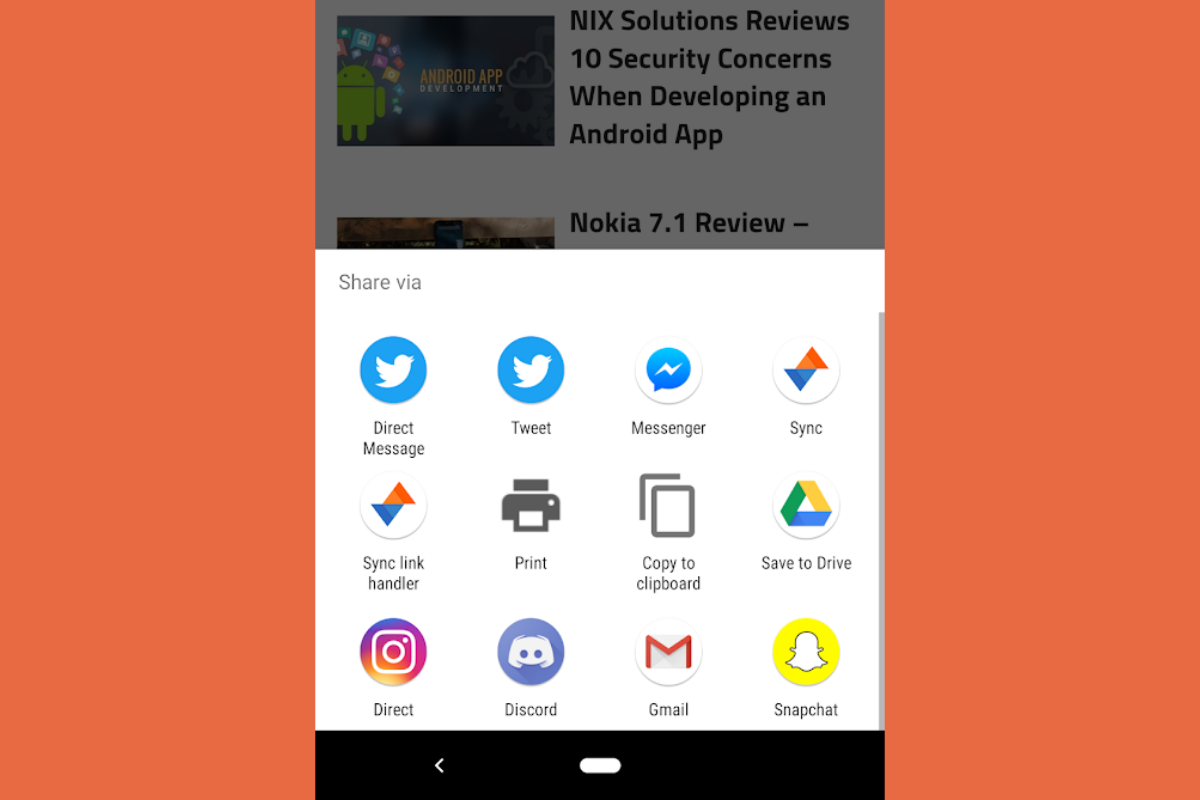The image portrays a screenshot taken on a smartphone, capturing a small pop-up window that occupies approximately half of the screen. This window, which appears as a white square, contains various sharing options. At the top left corner, the text "Share via" indicates the purpose of the window. Below this text, there are 12 icons arranged in a grid format, each representing a different method to share content.

Starting from the top left, the icons are as follows:

1. **Bird icon labeled "Direct Message"**
2. **Bird icon labeled "Tweet"**
3. **Messenger icon**
4. **Sync icon**
5. **Sync icon (repeated in the next row)**
6. **Print option**
7. **Keyboard shortcut**
8. **Save to Drive option**
9. **Instagram sharing icon**
10. **Discord sharing icon**
11. **Gmail icon**
12. **Snapchat icon**

Surrounding the pop-up window, the sides of the smartphone screen display a gradient background transitioning from light to dark red. This image showcases a detailed view of the phone's screen sharing interface, providing a variety of social media and utility options.